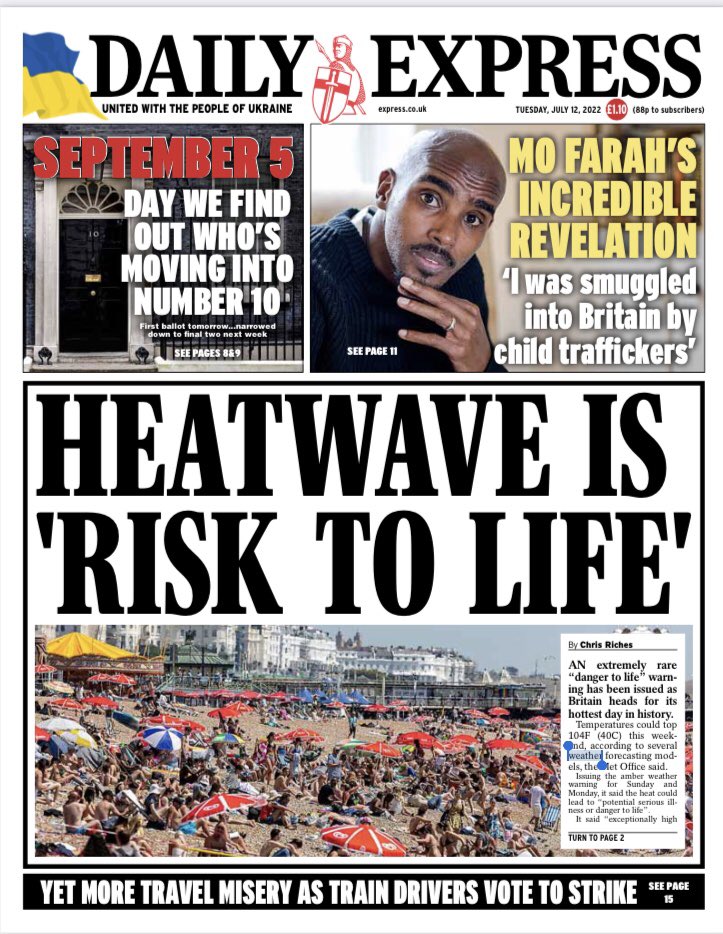This is an image of the front cover of a British tabloid-style newspaper called the Daily Express, dated September 5, 2022. Prominently featuring a variety of sensational news stories, the headline centers on a heatwave being a "Risk to Life," with a large, bold black font. Next to this, Mo Farah reveals, "I was smuggled into Britain by child traffickers," with his incredible story highlighted in a mix of gold and white text. Additionally, the paper mentions, "The day we find out who's moving into Number 10," indicating political news. In the top-left corner, there is a Ukrainian flag with the phrase "United with the People of Ukraine," symbolizing solidarity. The front page also features multiple photographs, including images of crowded beaches, suggesting a summertime setting. A smaller section at the bottom notes that "drivers vote to strike," and various other stories are interspersed across the page. The text at the top and many headlines are predominantly in black, while some dates and specific tags are in red. A knight's shield logo accompanies the title, adding to its tabloid appeal.